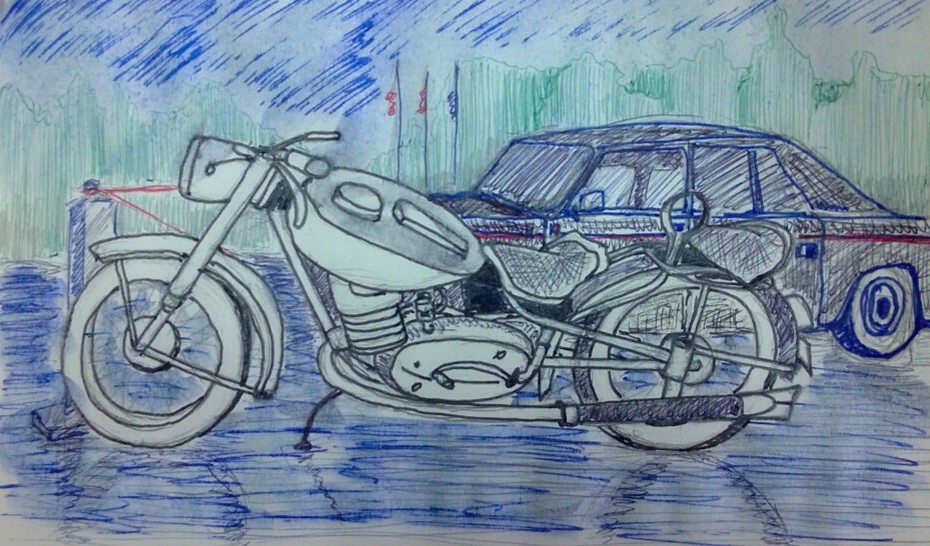The image is a detailed colored pencil drawing depicting a vibrant scene. In the foreground, there's a prominently drawn, sleek black motorcycle, resembling a V-twin type with big fat white-walled tires and a large headlamp. The motorcycle appears to be partially covering the front bumper of a four-door sedan, which is rendered primarily in black with blue trim and a distinctive red stripe. Both vehicles are parked on a road colored with blue lines and black accents.

In the background, a picturesque blue sky stretches across the top of the drawing, with a tree line spanning from left to right beneath it, represented by green lines. Above the tree line, three flagpoles rise, each topped with a flag in various hues of red and blue, adding a patriotic flair to the scene. The road and vehicles are complemented by the intricate details and bold color contrasts, capturing the viewer's attention towards the focal points of the piece.